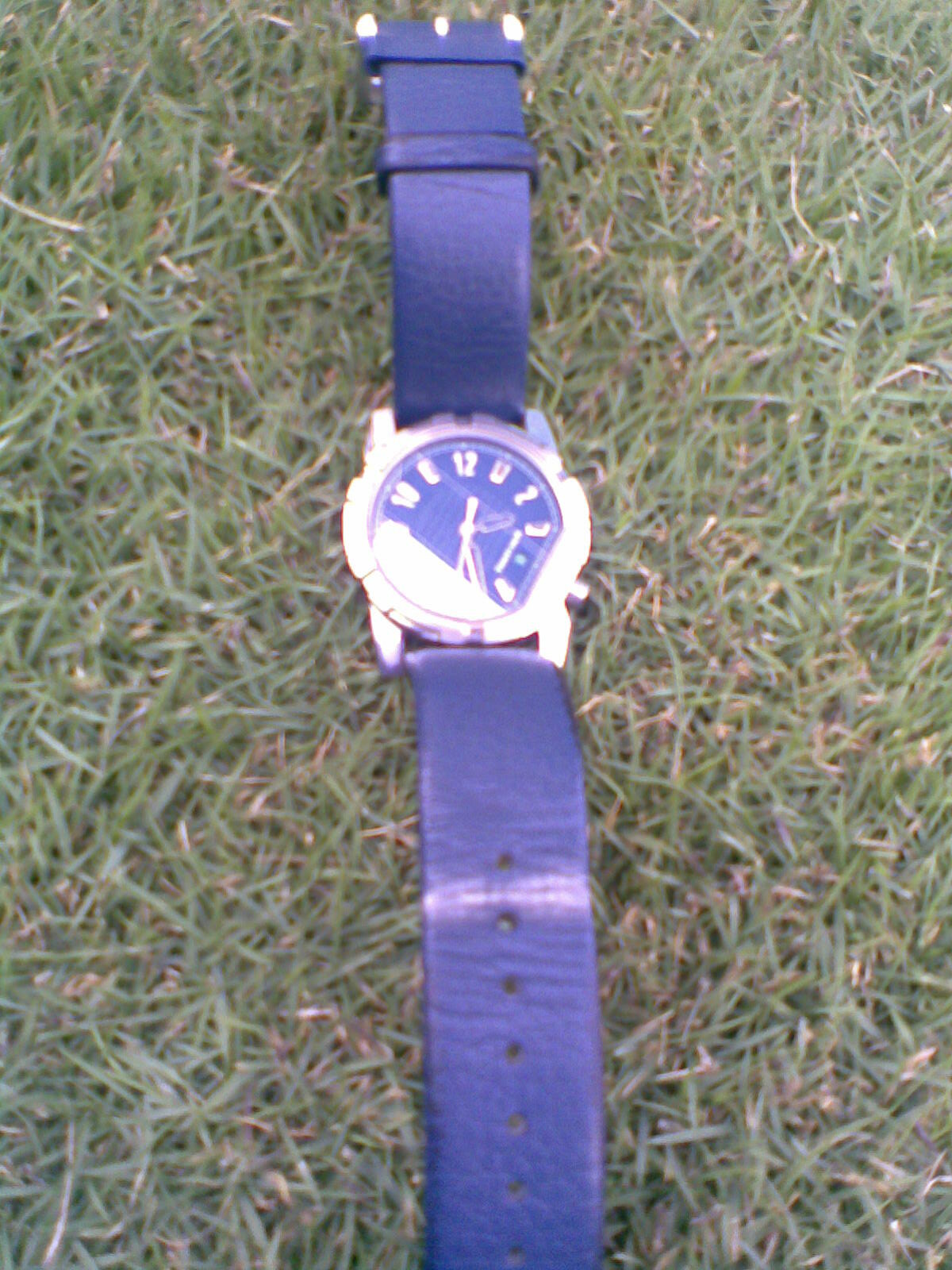The image features a wristwatch resting on a bed of lush green grass. Though the watch is somewhat blurry, its distinguishing features are still visible. The wristwatch sports a blue leather band, fully extended with the clasp and tongue in view, while the tail end, perforated with adjustable holes, is slightly cut off at the edge of the frame. The watch face catches an intriguing reflection of a building against the sky, making it challenging to discern at first glance. However, the watch face displays standard Arabic numerals for the hours, and the time shown is nearly 2:30, specifically around 2:26 or 2:27.